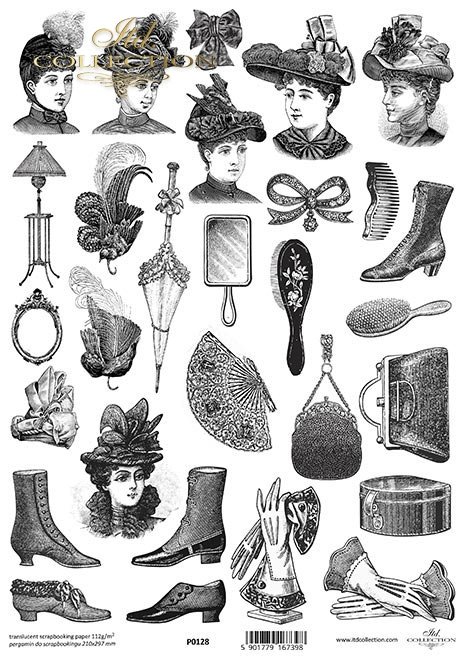The image is a detailed collage that appears to depict 19th-century women's fashion. At the top are five black and white illustrations of women, showcasing ornate, large hats and formal wear. Below these illustrations, various fashion accessories are scattered, including hand fans, umbrellas, boots, hairbrushes, mirrors, gloves, purses, and belts. Additionally, there are items like a lamp, and a bow. The image is primarily black and white with shades of gray, and includes subtle gold text that reads "The Collection" in the bottom right corner. A barcode is present, suggesting that these items might be part of a catalog or packaging, potentially for scrapbooking materials. The overall style and detailing hint at a late 19th-century aesthetic, reminiscent of an old magazine or catalog for women's fashion and accessories.